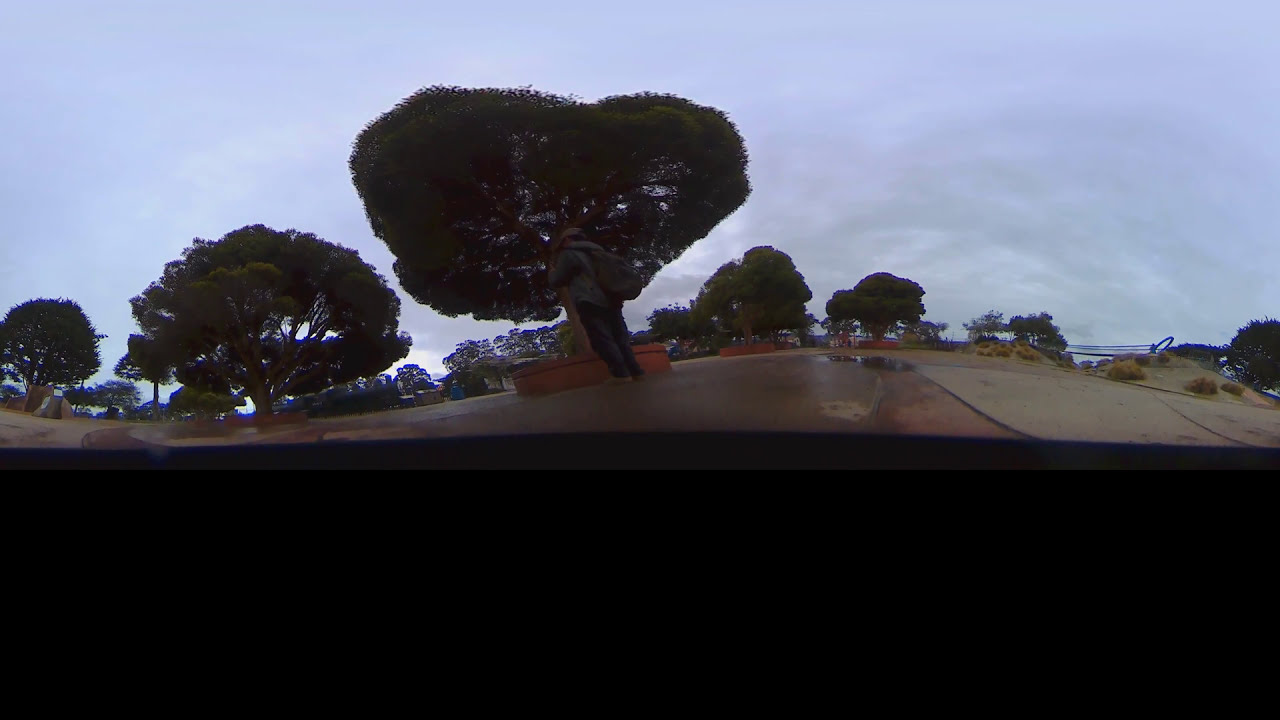In a park setting, a man stands prominently in the middle of the scene. He is attired in brown shoes, navy blue jeans, a gray jacket, and carries a gray backpack. The image, taken with a 360-degree camera, presents a wavy, sine-wave distortion that stretches across the gray, wet pavement beneath his feet, making the surface appear as though it's undulating. The park features wide, well-maintained trees planted in large, terracotta-colored planters that line the pathways. These trees are short yet have very wide trunks, giving them a robust and imposing presence with lush green foliage. The overcast sky blankets the scene in a muted light, suggesting recent rain, and the horizon hints at the presence of water in the distance. The overall atmosphere is gloomy, with a dark area covering the lower portion of the image, possibly from inside a vehicle or due to the way the image was cropped.